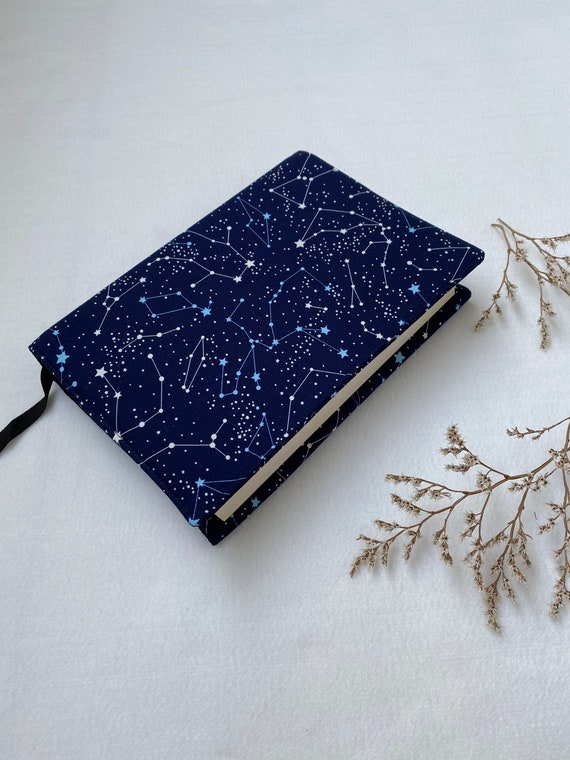The image features a thick, dark blue journal with a constellation theme, detailed with white stars and constellation lines. A black cloth bookmark peeks out from its pages. The journal rests on a white background, accentuated by brown twigs placed to the right for decorative purposes. The pages of the journal are white, and despite being closed, it suggests a well-crafted design suitable for writing, likely aimed at being sold on a shopping site. The colors on the cover combine dark blues, whites, and blacks, with some tan shades, showcasing a night sky motif.